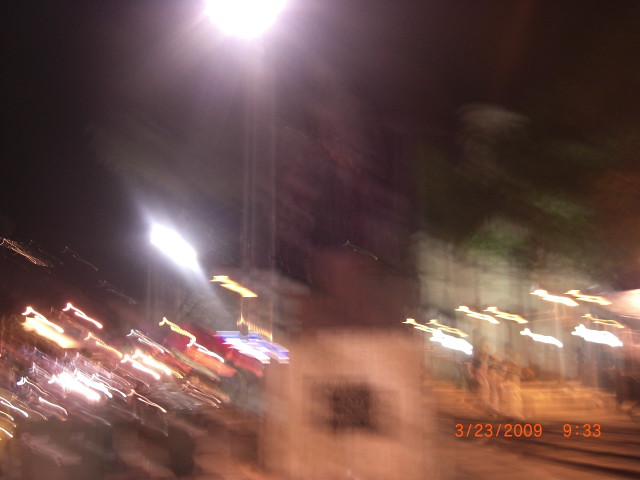A heavily blurred photograph capturing an indistinct scene suffused with an array of colors. Dominating the top center portion is a bright light casting a prominent glare downwards, illuminating what could be a road, a street, or an arena—it’s difficult to discern due to the blurriness. The image is awash with colors such as red, orange, blue, and white, with a noticeable brown at the bottom. Amid the unclear surroundings, two lights are reflecting within the frame, contributing to the overall haziness. In the bottom right corner, there is a clearly visible timestamp in orange, reading "3-23-2009-9-33," offering the only clear detail in this otherwise nebulous visual.